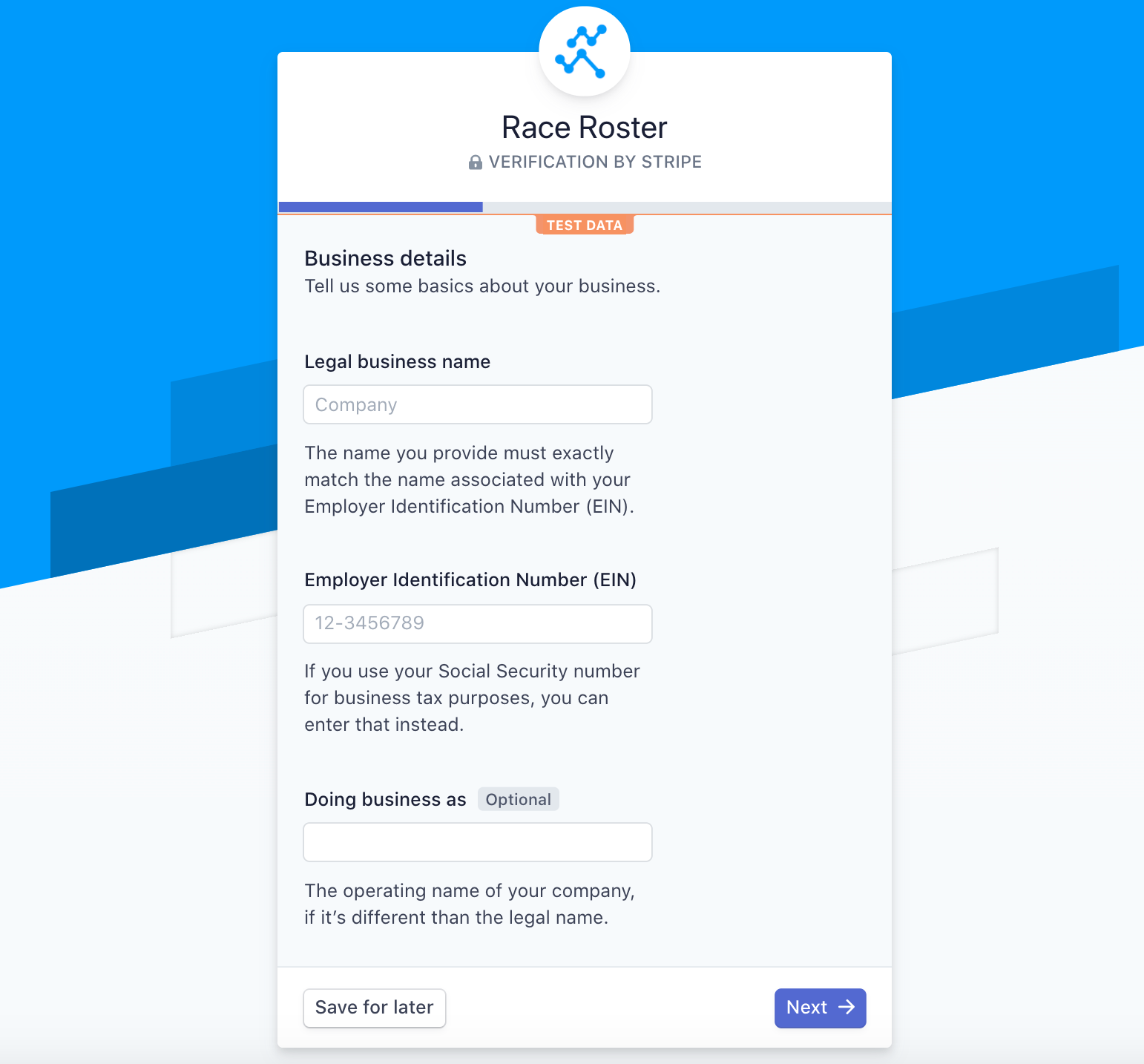The image features a user interface on a light blue background, with two darker blue sections at the bottom. A prominent white notification screen, possibly a pop-up, appears in the center. At the top of this screen is a circle containing a blue icon depicting stylized, curvy lines resembling a person running. Below the icon, the text "Race Roster Verification by Stripe" is displayed.

An orange box labeled "Test Data" is situated underneath this heading. The main section is titled "Business Details" and includes the instruction "Tell Us Some Basics About Your Business." There are two fields provided: "Legal Business Name," accompanied by an input box labeled "Company," and a disclaimer stating, "The name you provide must exactly match the name associated with your Employer Identification Number, your EIN."

Further down, a section for "Employer Identification Number, EIN" includes another text input box, along with guidance that "if you use your Social Security Number for business tax purposes you can enter that instead." Lastly, the form offers an optional section labeled "Doing Business As," with a corresponding input box. Instructions clarify that this should be used for the operating name of the company if it differs from the legal name.